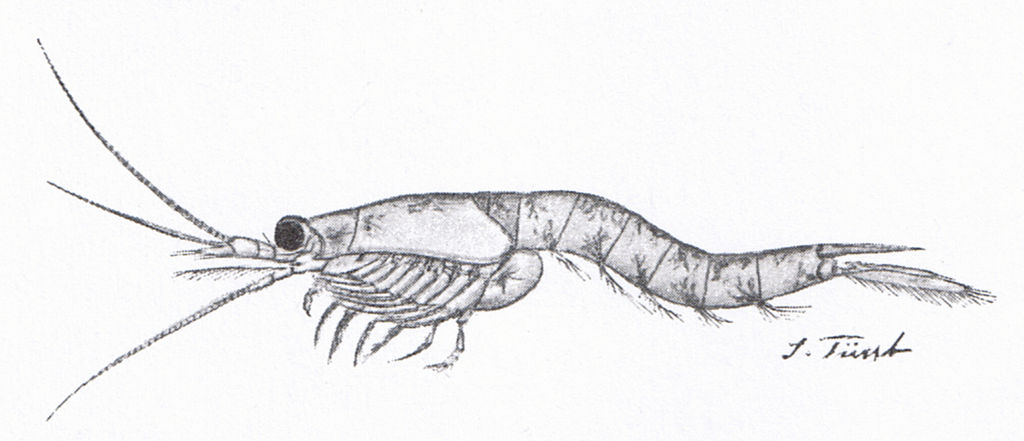This is a detailed pencil sketch of a shrimp, showcasing its intricate features in a side view as it faces left. The hand-drawn image, not a photograph, is rendered in black and white using graphite, giving it a range of gray tones with some effective shading to highlight its form. The shrimp has seven legs that vary in length, with those at the back being longer and those at the front shorter. These legs cluster near the shrimp's chest and close to its big, singular black eye. Three antennae extend from the front of its mouth, adding to the detailed anatomy portrayed. The body also features small hairs around the tail and underneath, enhancing the sketch's realism. The sketch is set against a white background and has an accurate depiction, capturing the likeness of the subject matter. Below the image, an artist's signature appears, reading "J. tint" or something similar. The drawing includes subtle dark gray spots that might resemble smudges, adding texture to the sketch. Overall, the artist's work is both precise and true to the appearance of a shrimp.